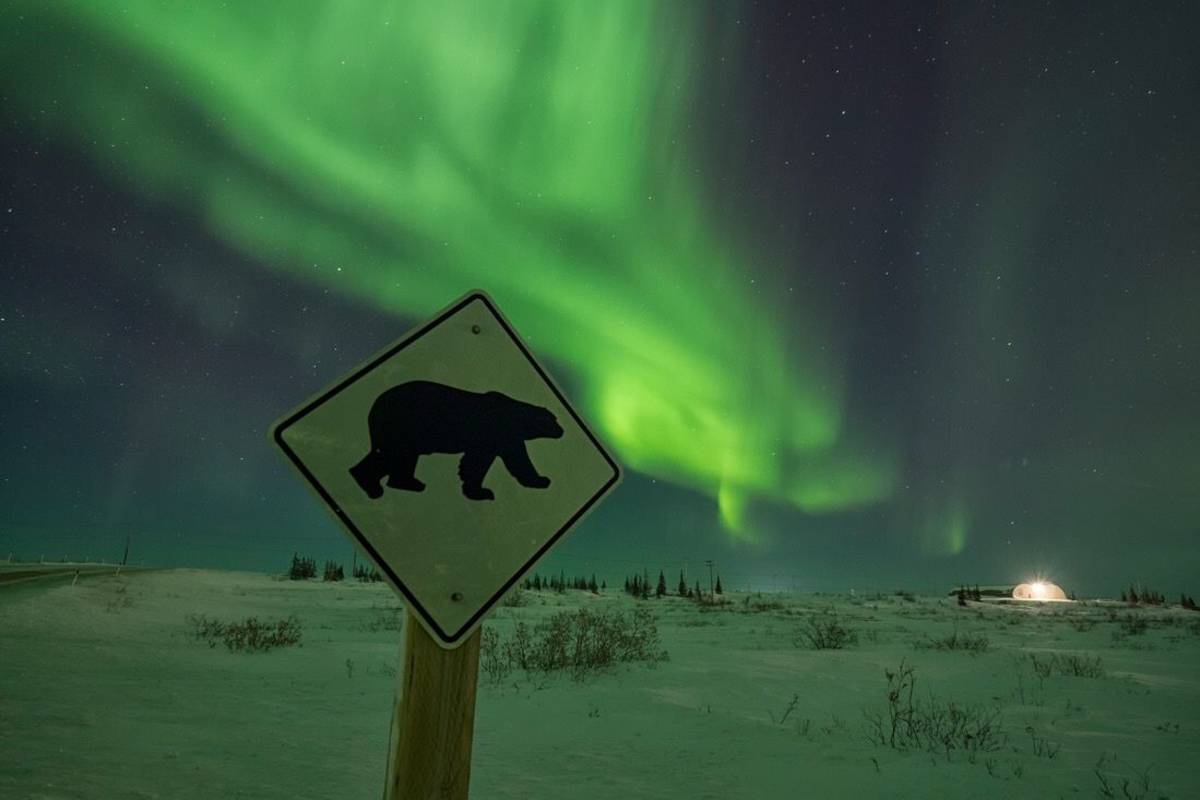In this captivating nighttime photograph, the forefront is dominated by a wooden post bearing a diamond-shaped, white sign with a striking black bear illustration, presumably a warning for bear crossing. Surrounding this post is a vast, snow-covered plain that stretches to the horizon, where a few scattered shrubs and distant trees are visible. The night sky overhead is a mesmerizing display of the Aurora Borealis, predominantly green with hints of yellow, casting a surreal glow over the landscape. The deep blue of the night sky, dotted with white stars, adds to the ethereal ambiance. In the distance, to the right, there is a brightly lit dome structure, possibly an Eskimo house, its light shining prominently in the otherwise barren and serene environment. To the left, a small road meanders through the terrain, enhancing the scene’s remote and tranquil feel.